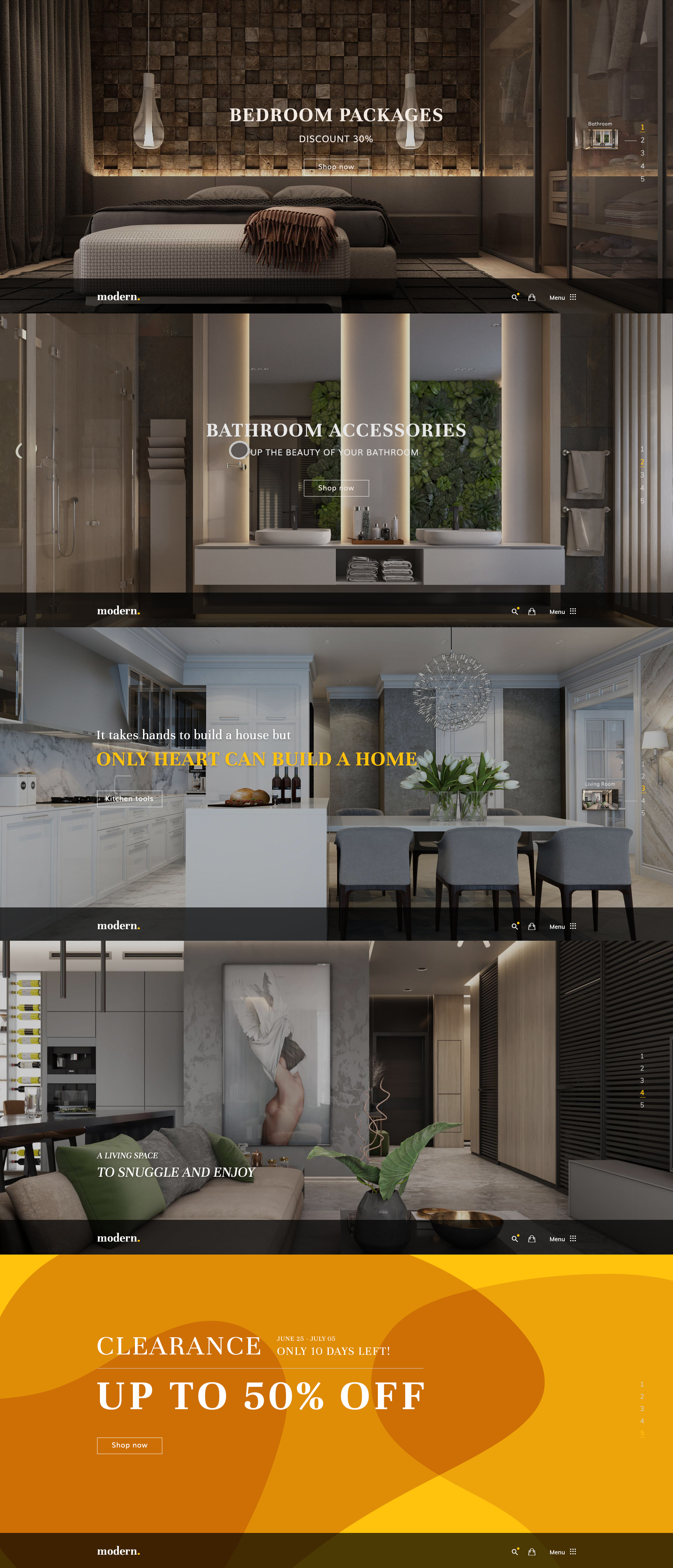The image is a composite of several promotional visuals stacked vertically, each representing different home environments with accompanying text and design elements that convey a luxurious lifestyle. 

At the top, the first image advertises a "Bedroom Package" with elegant white text superimposed on a scene of a lavishly decorated bedroom, complete with rich textures and sophisticated furniture.  

Beneath it, the second image promotes "Bathroom Accessories," displayed in the center using white font over an image of a chic and opulent bathroom, highlighting stylish fixtures.

The third image showcases a kitchen, featuring the phrase "Only Heart Can Build a Home" in prominent yellow lettering. The kitchen is depicted as both modern and inviting, emphasizing the warmth and care that make a house a home.

Following that, the fourth image presents a luxurious lounge area, with cozy furnishings and a warm ambiance. White text on this image invites viewers to "Snuggle and Enjoy," perfectly capturing the comfort of the space.

The final image features a vibrant yellow and orange gradient background with a prominent "Clearance" sign, advertising discounts of up to 50% off. A "Shop Now" button is located on the left-hand side, urging immediate action from the viewer.

Each of these images includes a small grey panel at the bottom left corner with the word "Modern," subtly branding the content. This panel appears consistently across all images, reinforcing the identity of the website or brand being advertised.